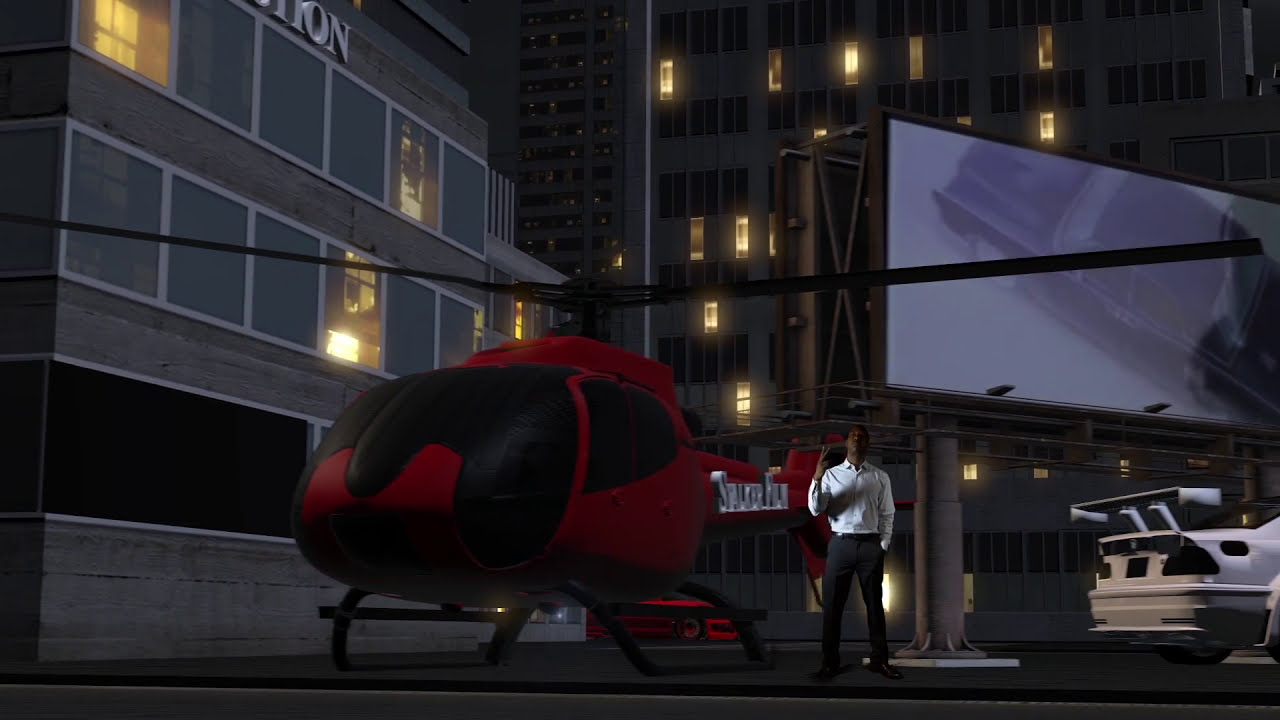The horizontally aligned rectangular image, resembling a screenshot from a video game, depicts a nighttime scene on a helicopter pad. Centered in the image is a red and black helicopter with its black blades visible. To the right of the helicopter stands a man in a white button-down shirt and grey pants, with his right arm raised in a victory sign and his left hand in his pocket. Behind the man, slightly to the right, is the back end of a white sports car with a high spoiler. The setting includes two multi-story buildings; the one on the left appears to be a two-story brownstone, while the one on the right, partially cut off at the top, reveals several lit windows. There’s also a prominent display screen behind the man, featuring an image of a car on a road. Above the left building, grey letters spell out "T.O.N." in an upper segment, adding to the details of the scene.